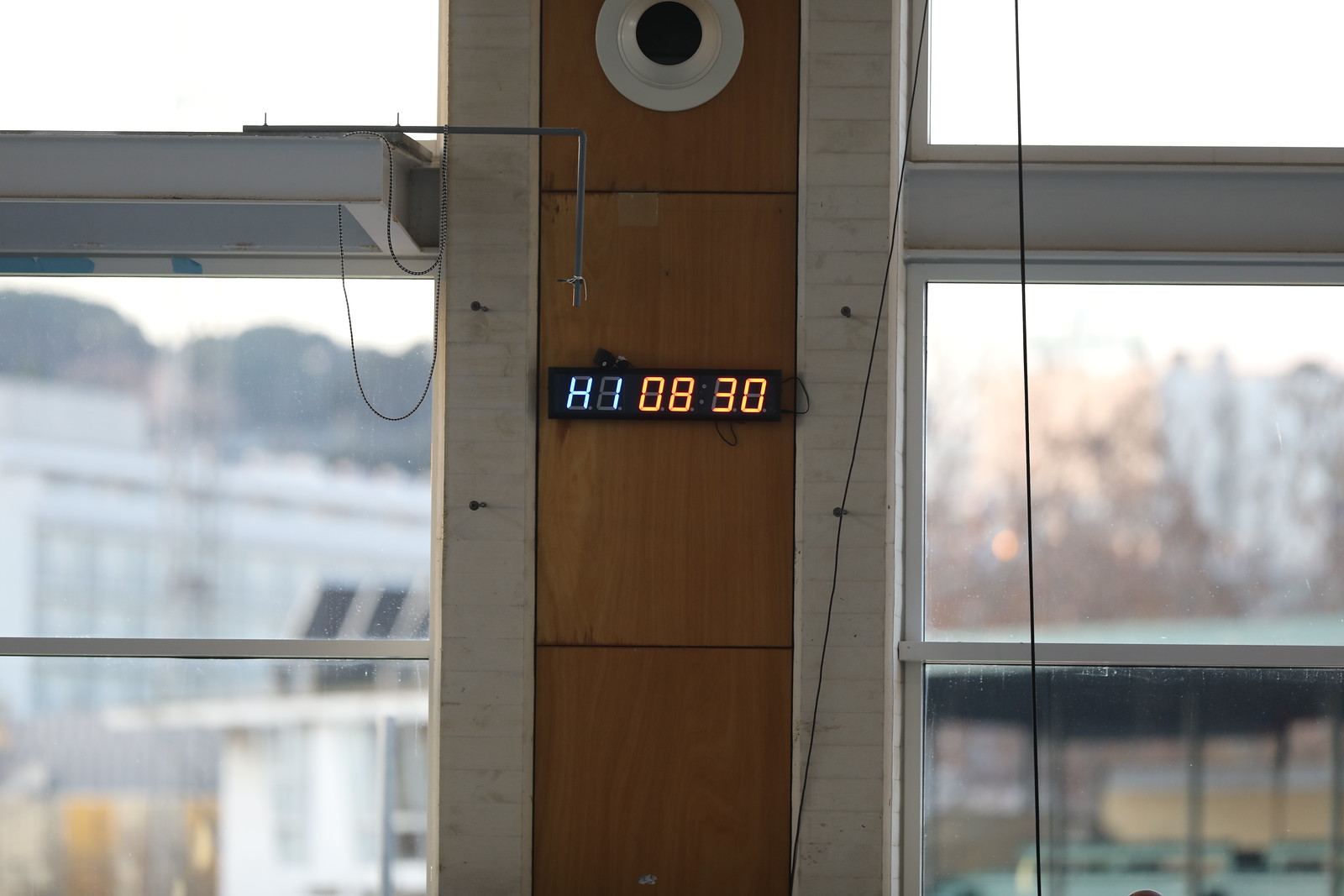This detailed daytime interior photo features a brown wooden column positioned centrally against a wall, flanked by two aluminum-framed windows. The windows consist of two visible panes each: a lower double pane and an upper single pane. The exterior view through the windows is vague and blurry, revealing indistinct shapes of buildings, trees, and vehicles. The column, divided into three sections with gray-tiled edges, occupies the center from the bottom to the top of the picture. 

Mounted on this wooden pillar is a thin horizontal digital screen displaying 'HI 0830' - 'HI' in light blue and '0830' in orange. Above the screen, at the top of the column, a round white circular frame with a black dot in the center is visible, which looks like it could be a camera. Additional details include a hanging metal rod and wires visible above the digital display.